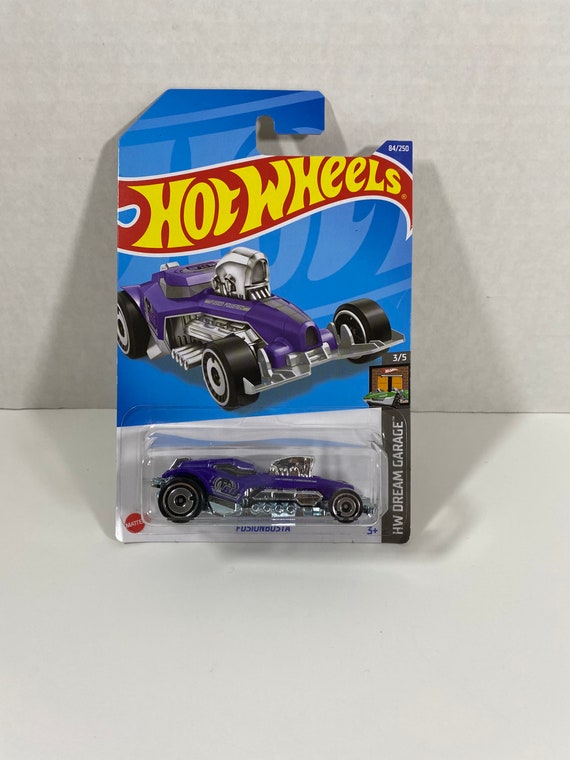This image shows a Hot Wheels toy car still in its packaging, placed on a white table against a white background. The iconic Hot Wheels logo, in bold yellow letters with a red flame graphic and white trim, adorns the top of the blue cardboard backing. The car, encased in a clear plastic shell, is prominently displayed underneath. It is a purple muscle car with black wheels, featuring a large, mean-looking engine protruding from the hood. Just below the car, the name "Fusion Gusta" is inscribed, and the label also indicates an age rating of "3+".

On the lower left corner of the package, the Mattel logo is visible in a red circle with white text. The package also has "84/250" written in small white text at the top right corner. Vertically aligned on the left side is the label "HW Dream Garage," accompanied by a small Hot Wheels flame logo and the fraction "3/5." This detailed and colorful display exemplifies the classic Hot Wheels design and packaging.